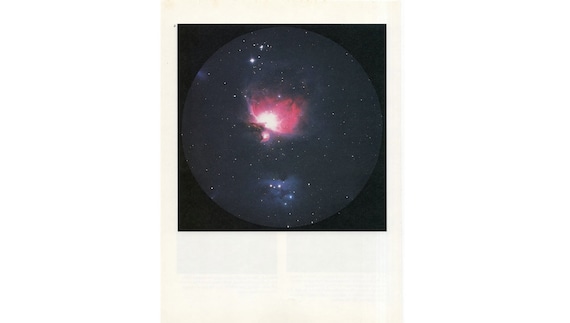This image features a vintage-style Polaroid photograph with a classic white border, where the bottom part is slightly larger than usual and contains faint black rectangular markings. The main focus of the Polaroid is an astronomy-themed digital rendering showcasing a celestial scene. At its center is a circular formation resembling a gas giant or an irregularly shaped galaxy with a red-orange core that gradually fades into pinkish hues towards the edges. The formation is dotted with multiple bright white projections, mimicking stars, and accented with subtle blue highlights on the upper left and lower center portions. The circle is centrally positioned against a black background, adding depth and emphasis to this captivating outer space image.